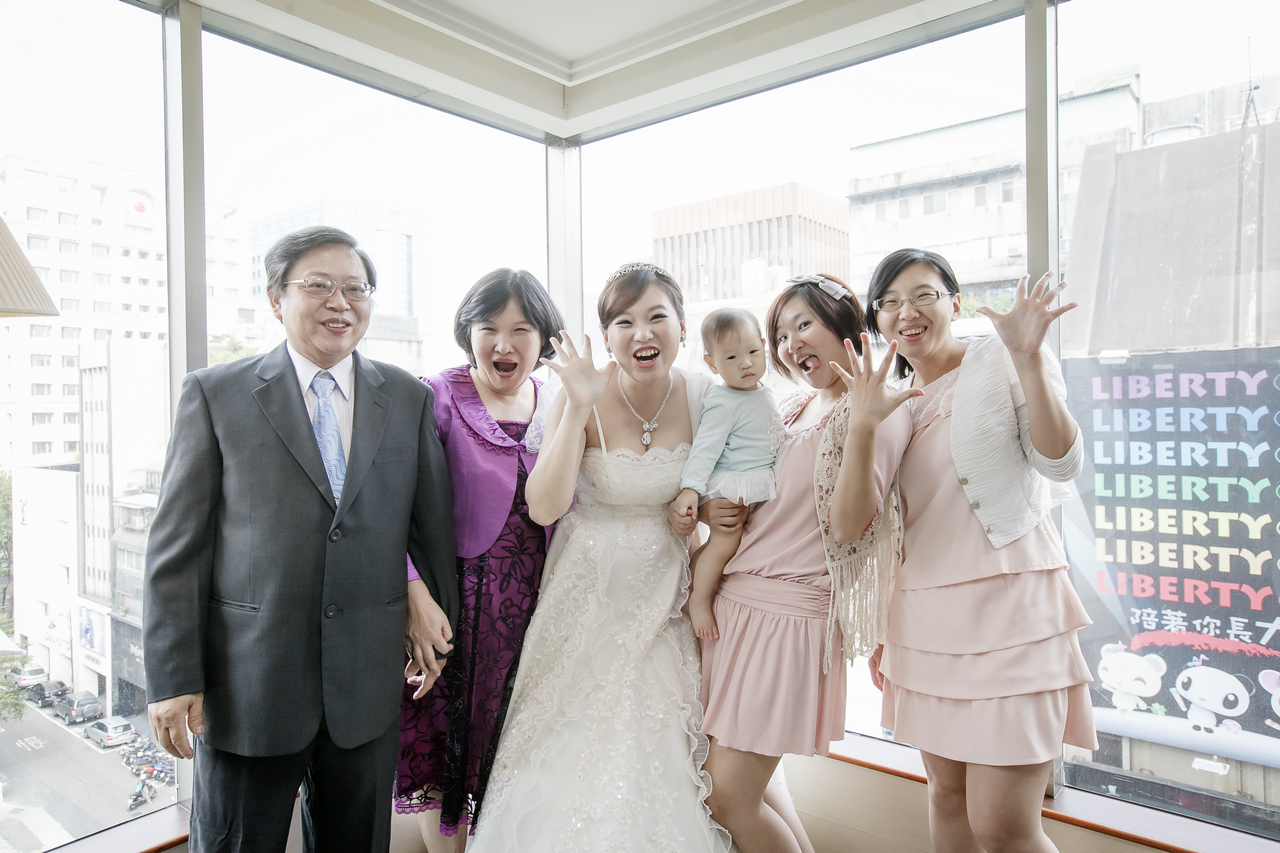In this vibrant photograph, we see a joyful wedding scene set inside a bright, airy venue with large windows offering a view of neighboring buildings. At the center of the image stands a radiant bride, dressed in a beautiful, elegant gown, exuding happiness on her special day. To her left, an older man beams with pride, while on her right, an older woman shares in the joy alongside her. Adjacent to the older woman, a younger woman stands tall, accompanied by two other women, one of whom is gently cradling an unimpressed baby. The surrounding women are cheerful, with some striking playful poses, adding to the fun and celebratory atmosphere of the moment. Their outfits complement each other with frilly designs, creating a harmonious visual ensemble as they celebrate the union of the radiant couple.